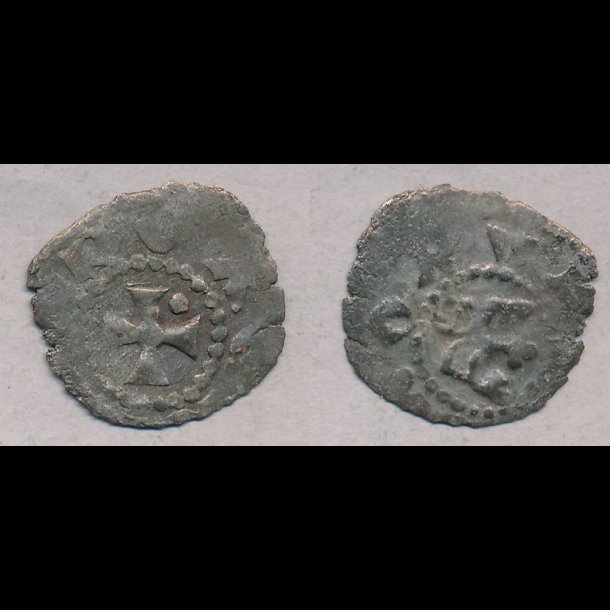This highly detailed photographic image features a central light gray panel bordered by two thick black panels at the top and bottom. Displayed on the panel are two ancient-looking, round, silver coins with rough, gouged edges, indicating significant age and wear. The coin on the left showcases a cross design made up of four triangles, encircled by a dotted border. The coin on the right presents an intricate script at its center, surrounded by concentric circles, though the script is mostly illegible and doesn't appear to be in the Roman alphabet. Both coins sit on a white background that contrasts sharply with the surrounding black panels, enhancing their weathered and historical appearance.